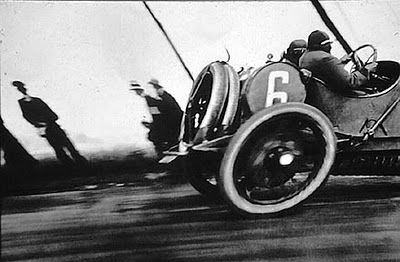This black-and-white photograph vividly captures a vintage race car, actively engaged in a race. The car, designated with the number six, showcases an open carriage design devoid of a roof, and is equipped with two spare, narrow tires mounted on the back. The image exudes an antiquated essence, accentuated by the distorted appearance, perhaps caused by the camera's attempt to capture the motion of the speeding vehicle. This distortion renders the background slightly blurred, giving an impression of speed and movement. The setting appears to be a race track or road, with a slick, dark surface that might be wet or oily. In the background, several figures are discernible, including a man who resembles a policeman, and two men and two women walking. The grayscale tones of the photograph enhance the nostalgic atmosphere, making it a compelling snapshot of an era long past.